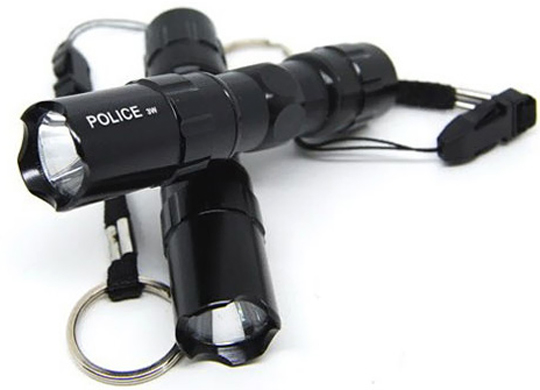This image captures a pair of black, handheld police flashlights displayed against a completely white background. Each flashlight, ergonomically designed for a comfortable grip, is made of substantial metal and measures about six inches in length. The flashlights are positioned one on top of the other, with their lenses facing the viewer. The top flashlight prominently features the word "POLICE" in white capital letters, followed by "TM" indicating its trademark status.

Both flashlights are equipped with black lanyards attached to their ends. One lanyard includes a silver split ring keychain, while the other is clipped together with a black clip. The lanyards, detailed with braided black thread, offer convenient options for attachment to a belt or key ring for easy access. This detailed arrangement hints at the flashlights being part of a purchasable display, highlighting their use and design features.